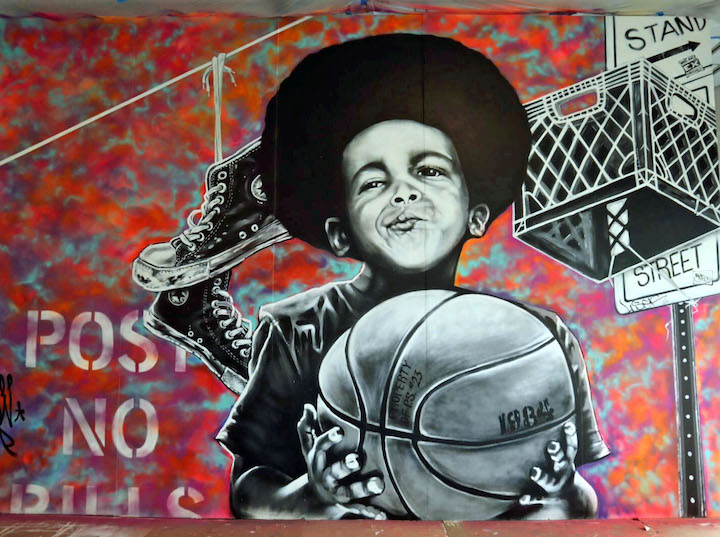The image, resembling a mural or graffiti art, centers on a young African-American boy, around 10-12 years old, standing proudly while holding a basketball marked with "1984" and "PS 23." He has a black Afro and wears a black shirt. The boy and his surroundings are depicted in black and white, including a pair of Converse shoes dangling by their laces from a line and a milk crate repurposed as a basketball hoop attached to a street sign. The sign reads "Stand" with "Street" below it. The colorful background features a blend of light blue, orange, pink, purple, and some specks of red and green, contributing to the graffiti-like aesthetic. In the bottom left corner, partially visible text reads "Post No." and another obscured word.